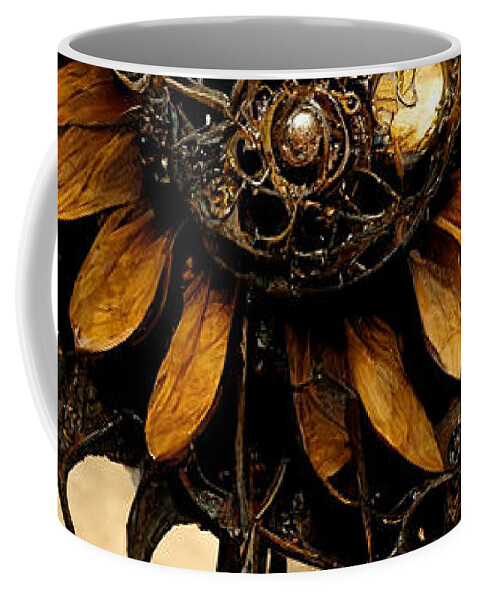This image depicts a mug set against a plain white background, giving it a stark, stock-photo feel. The focus is entirely on the mug, which features a white handle, interior, and top rim. The base of the mug showcases a darker, rustic design with intricate elements. Covering the exterior is a very zoomed-in floral pattern that appears to be a dead or decaying flower, with yellowish-brown petals that suggest either a dried or a fabric-like texture. The center of the flower bears a complex, somewhat medieval circular design, reminiscent of natural roots or an abstract ocular form. This is a captivating and enigmatic image with the mug's floral motif serving as the central visual element.